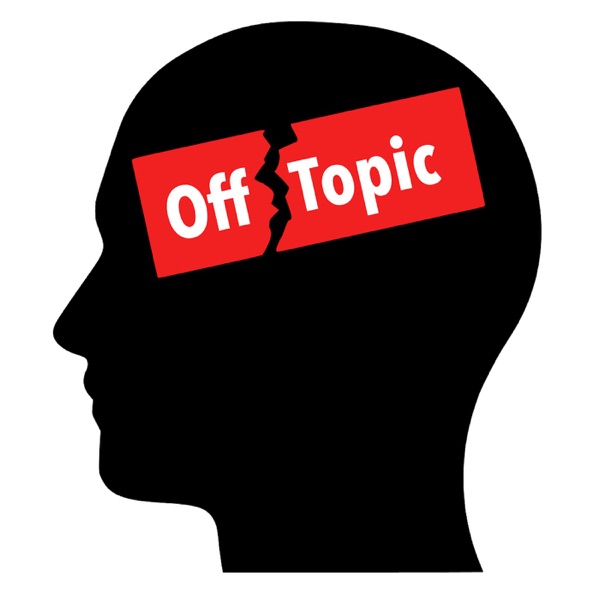The image depicts a digital creation centered on a plain white background, featuring the side profile of a human head in black silhouette. The profile, facing left, includes distinct outlines of the mouth, nose, and neck, and ends just below the chin. The silhouette is adorned with a horizontal red rectangle that spans from where the eyes would be to the back of the head, which appears to be jaggedly torn into two uneven sections. Inside this red rectangle, in white text, are the words "off topic" – "off" occupying the larger left portion and "topic" the smaller right portion. The minimalistic design, constrained to the colors white, black, and red, gives the impression of a company logo or an online graphic. The silhouette is large, taking up almost the entire space and is centrally positioned with the text predominantly in the upper region of the image.